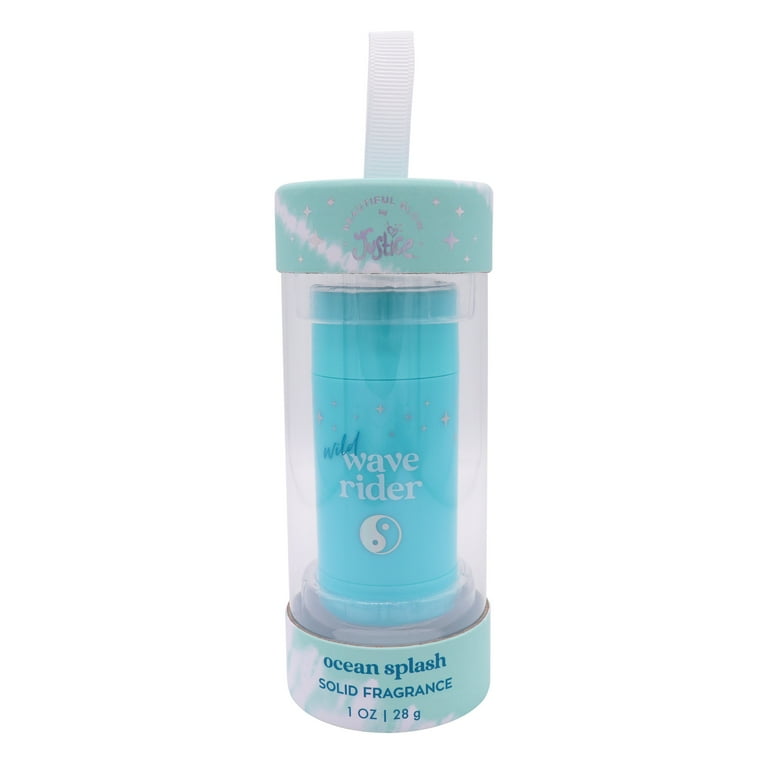The image depicts a product named Wild Wave Rider Ocean Splash Solid Fragrance housed in a distinctive plastic container resembling a drinking cup with a straw-like protrusion at the top. The container, primarily seafoam green with a clear front, reveals an inner blue container that looks similar to a deodorant stick. At the base of the container, in dark teal text, it states "Ocean Splash Solid Fragrance, 1 ounce, 28 grams." The inner blue container is labeled "Wild Wave Rider" and features a yin-yang symbol in white and blue. Above this, the cap of the container bears small, unreadable text in an arc, with the readable word "Justice," where the "I" is stylized as a heart. The straw emerging from the top appears slightly ribbed, suggesting it can be bent. The overall design conveys a clean and fresh aesthetic.